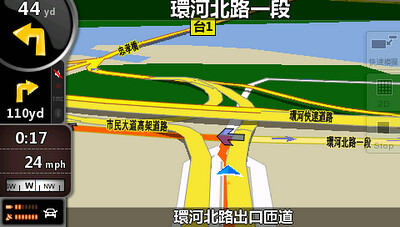This image captures a detailed screenshot of a GPS navigation screen, featuring various navigational elements and data in what appears to be Japanese at both the top and bottom sections. On the left side, directional arrows indicate the distance to upcoming turns, starting with a left-hand turn at 44 yards, followed by a right-hand turn at 110 yards. Additional details include a timer showing 17 seconds and a speed display of 24 miles per hour. The direction of travel is indicated as west. In the bottom left-hand corner, there are two light fixture icons alongside a car symbol, the specific meaning of which is unclear. The map displayed on the GPS screen reveals a complex network of highways, showcasing the intricacies of the road system being navigated.